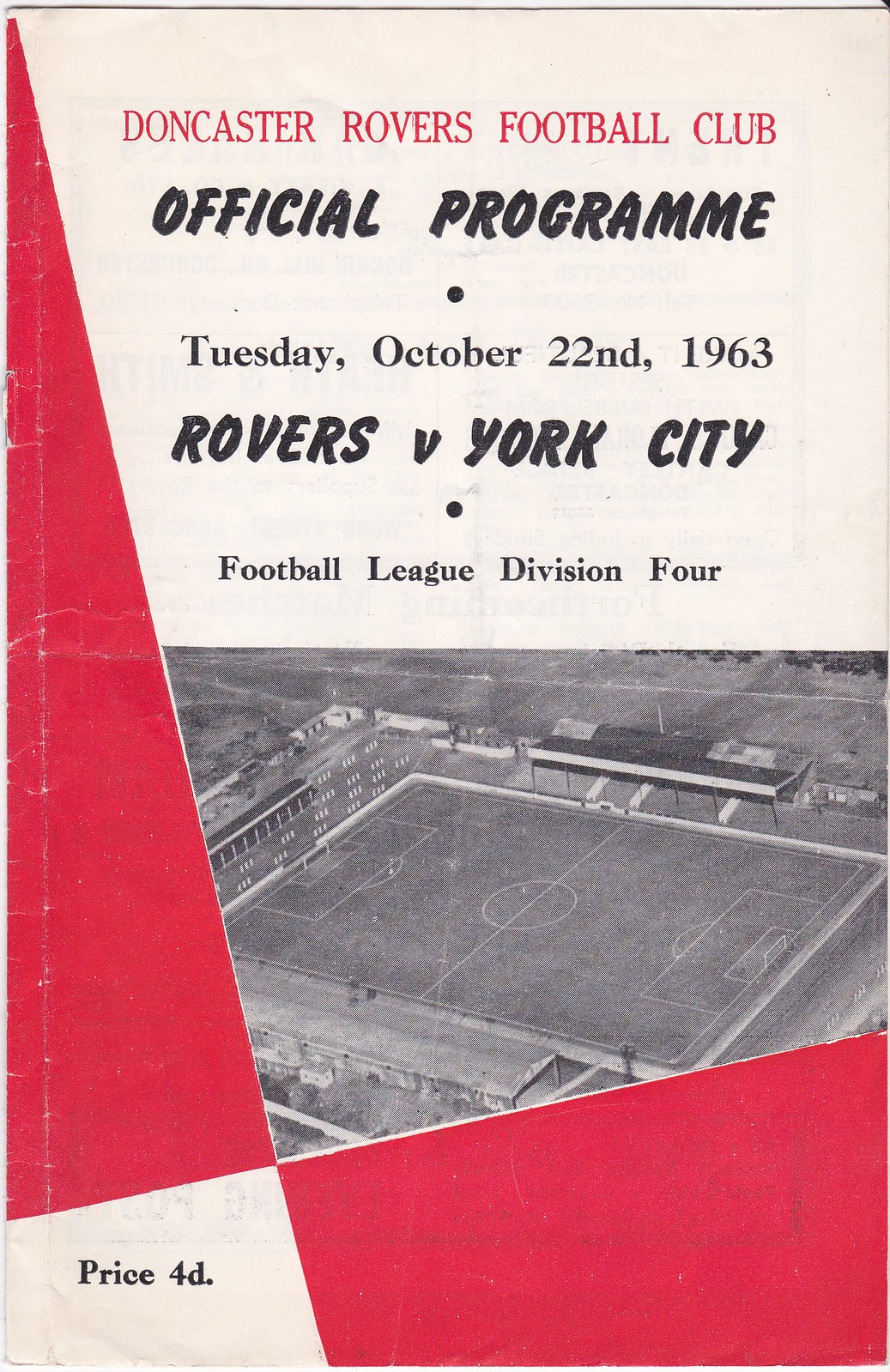This image depicts a worn and weathered official program from a soccer match. At the top of the program, set against a light cream background, "Doncaster Rovers Football Club" is prominently displayed in red letters within a white square. Below this, in bold black font, it reads "Official Program." Centered under this, the program specifies the date as "Tuesday, October 22nd, 1963" with a small dot on either side. The match-up is noted as "Rovers versus York City," followed by another center dot, and beneath that, it states "Football League Division Four." A large red triangle extends across nearly two-thirds of the page to the left. Dominating the center of the page is a black-and-white photograph of the soccer stadium where the event took place. In the very lower left corner, there is a small geometric white shape, while in the lower right corner, part of a red square is visible. Additionally, the price "4D" is noted just above the bottom left corner.